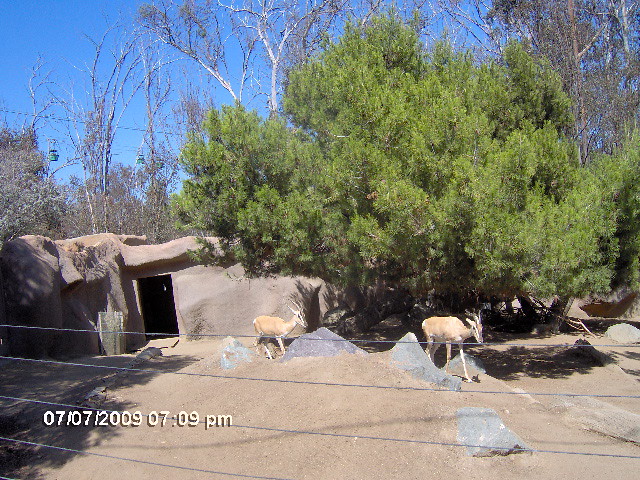This photograph, taken on July 7, 2009 at 7:09 PM, depicts an enclosure in a zoo under a vibrant, clear blue sky. The focal point is a large green tree surrounded by two sleek, beige-colored antelopes with black horns and white legs walking on a brown dirt path. They roam within a gray wire fence enclosure, bordered by jagged gray rocks and additional black rocks. To the left, fake rocks feature a human-made cave structure, possibly for the animals to sleep in. An overhead tramway with small carriages is visible in the distant background, adding to the zoo-like atmosphere. Other green trees with bare, beige branches stretch into the sky, indicating the enclosure may be seen during a dry season or maintained to appear this way. The date "07-07-2009" and time "07:09 PM" are stamped in white in the bottom left corner of the image.